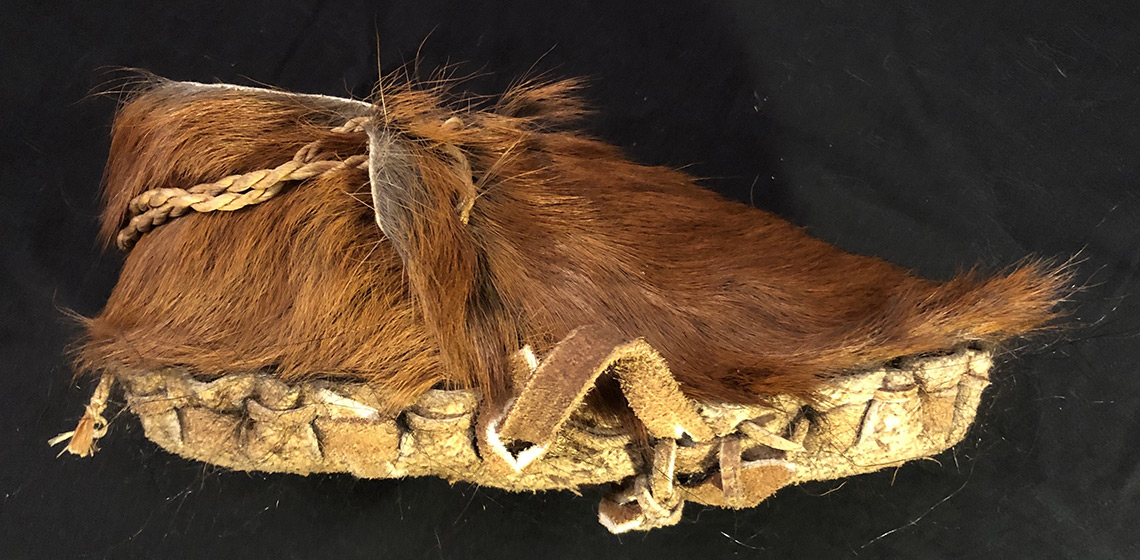The image showcases a detailed, horizontal, rectangular picture of what appears to be a primitive moccasin or slipper, possibly inspired by Native American footwear, centered on a black marbled background with some gray on the upper right side. The well-lit moccasin, occupying nearly the entire image, is characterized by thick, medium brown fur resembling that of a brown bear or horse, with a gradient from dark brown at the front to lighter brown at the back. The base of the moccasin appears to be made from a rough, tan-colored rawhide, tied together with thin laces along the edges. This footwear features a short platform wrapped in rope, with additional rope intertwined near the top, and a part for the ankle on the left side, sloping downward toward the front. A small, hard-to-read white tag with brown or black lettering is embedded within the fur, adding an element of authenticity to this museum-like artifact.